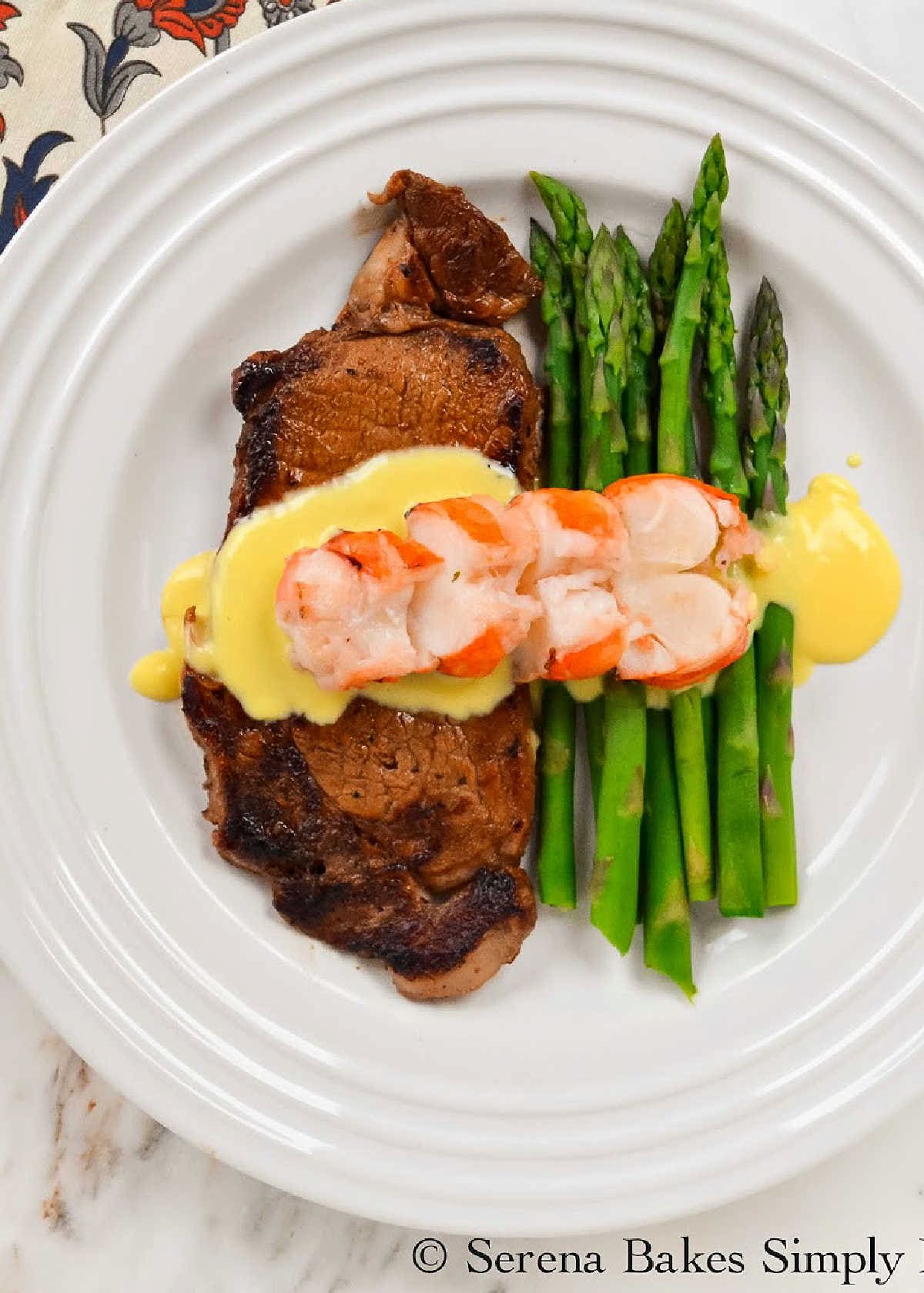This overhead photograph captures a meticulously arranged dinner plate sitting atop a marble-like countertop. The round, white plate showcases an elegantly seared piece of meat on the left side, likely a pork fillet given its lighter color and charred edges. To the right of the fillet lies a bundle of whole, vibrant green asparagus. Draped over the pork fillet, a succulent lobster tail adds a touch of lavishness, while a smooth, yellow sauce beneath adds an extra layer of flavor and visual appeal. A beige napkin with a floral pattern featuring gray leaves and red flowers peeks from the upper left corner beneath the plate. In the bottom right, text in black reads "Serena Bakes Simply," marking the image with an elegant touch. No other items clutter the clean, sophisticated presentation of this dish.